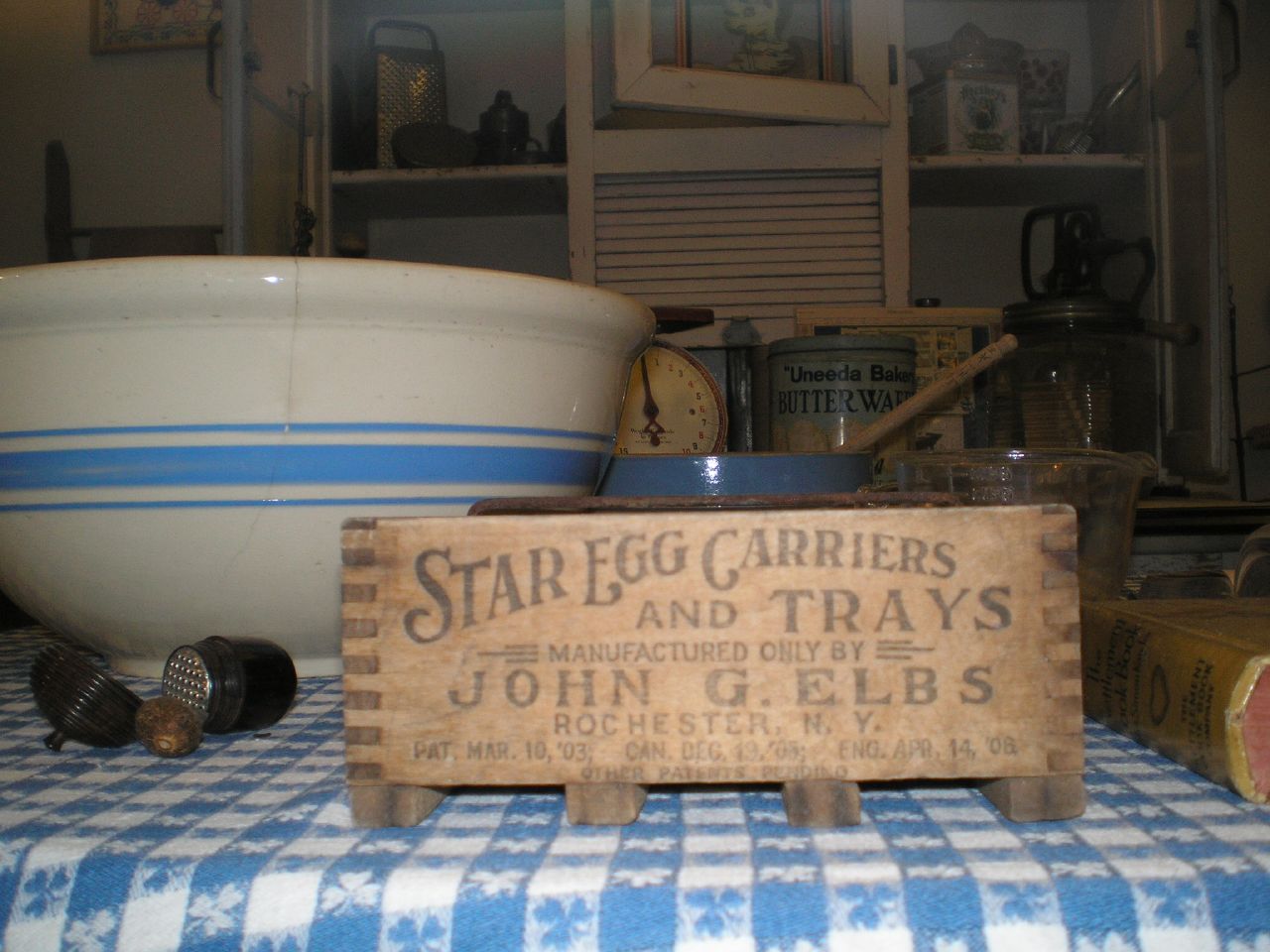This image showcases a nostalgic kitchen setup centered around a table adorned with a vertically striped blue and white tablecloth. Dominating the table is an aged wooden box elevated about an inch off the surface, inscribed with "Star Egg Carriers and Trays, Manufactured only by John G. Elbs, Rochester, New York," and displaying patent dates ranging from March 10th, '03 to various dates in 1905. To the left of the box, a large, round ceramic bowl, predominantly white with a broad blue stripe and two thinner blue stripes encircling it, sits prominently. Nestled beside this bowl appears to be another smaller, blue bowl containing a wooden utensil.

To the right of the wooden box rests a brown-covered book and a nearby glass jar. Behind the box, the backdrop features inset shelves cluttered with a variety of items, including a yellow-fronted vintage scale, a large jar, a tea kettle, and several canisters, one labeled "butter." Additionally, a black tool resembling a cheese grater or potato shredder is positioned next to a potato on the table. Salt and pepper shakers can also be spotted near the front of the large bowl. This detailed arrangement evokes a sense of timeless kitchen warmth and utility.